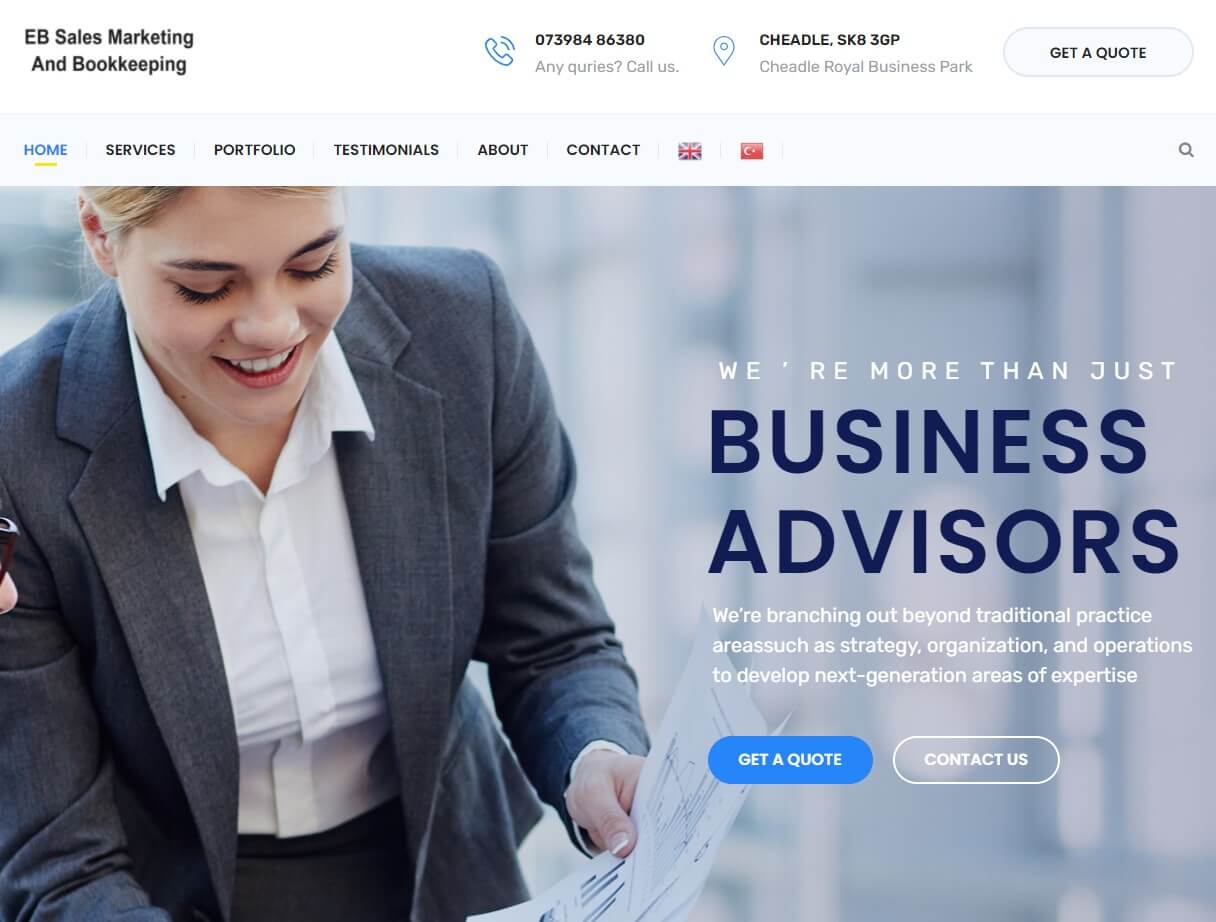In the upper left corner of the image, there is text in two lines that says "EB Sales Marketing and Bookkeeping". Moving across the image, you can see a blue telephone icon accompanied by a contact number, and below that, the location is stated as "Cheadle SK8 30P" at "Cheadle Royal Business Park". Below this, there is a prompt saying "Get a quote".

Dominating most of the page is a large picture of a fairly young woman with blonde hair neatly pulled back. She is wearing a grey blazer over a white dress shirt and is intently looking down at some sheets of paper.

Adjacent to the image, there is a statement: "We're more than just business advisors. We're branching out beyond traditional practice areas such as strategy, organization, and operations to develop next-generation areas of expertise. Get a quote or contact us."

Notably, there is a typo in the phrase "traditional practice areas such" since there is no space between these words.

At the top of the image, there is a navigation menu that includes the following options: "Home," "Services," "Portfolio," "Testimonials," "About," and "Contact."